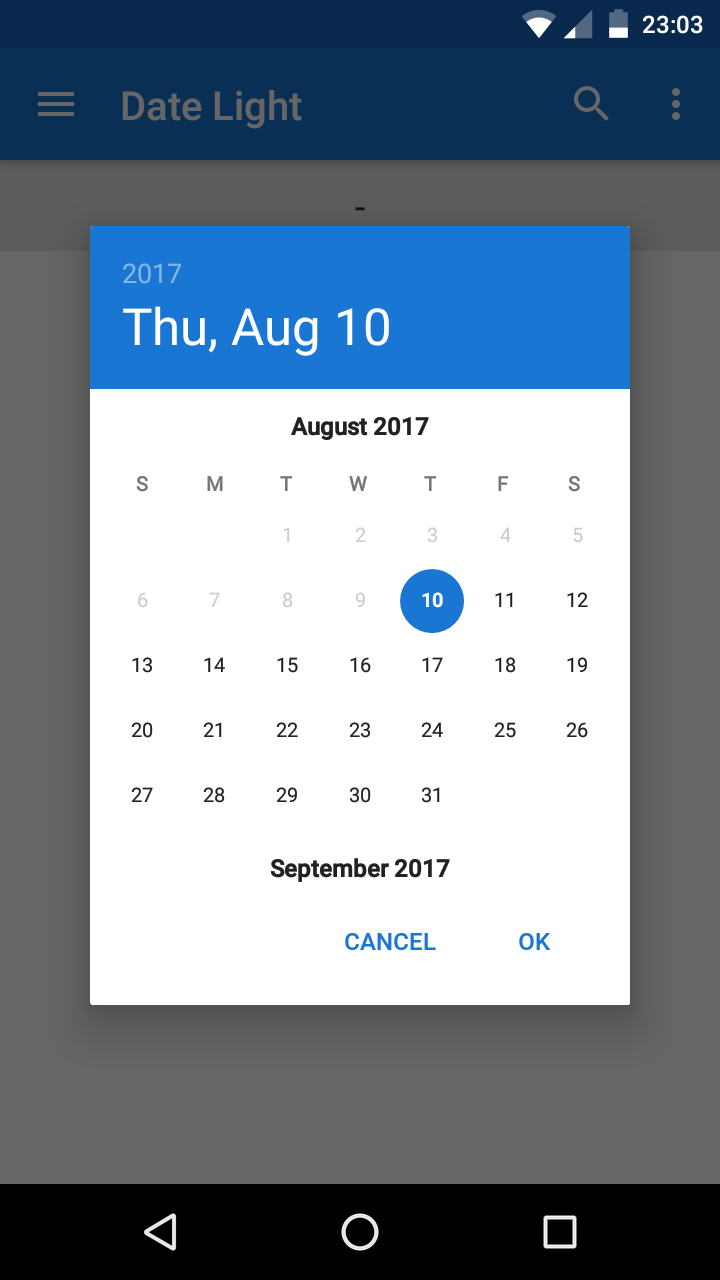A detailed screenshot captures a calendar scheduling interface on a smartphone. The main focus is a pop-up calendar overlay, displaying dates in August 2017. The background screen, dimmed for focus, features the text "Date Light," a search icon, a three-dot menu, and a hamburger menu at the top. In the top right corner, standard service icons for Wi-Fi, cellular signal, battery, and the time, which reads 23:03 (11:03 PM), are visible.

The pop-up calendar prominently highlights Thursday, August 10, 2017, as the selected date, which is also the current date of selection. Dates prior to August 10 are grayed out, while future dates appear in black text, indicating their availability. The header for September 2017 is also visible, though no specific dates for this month are shown. Below the calendar, blue text buttons for "Cancel" and "OK" are displayed.

At the bottom of the screen, the navigation bar includes three iconic buttons: a white triangle on the left, a circular home button in the center, and a square menu button on the right, all set against a black background.